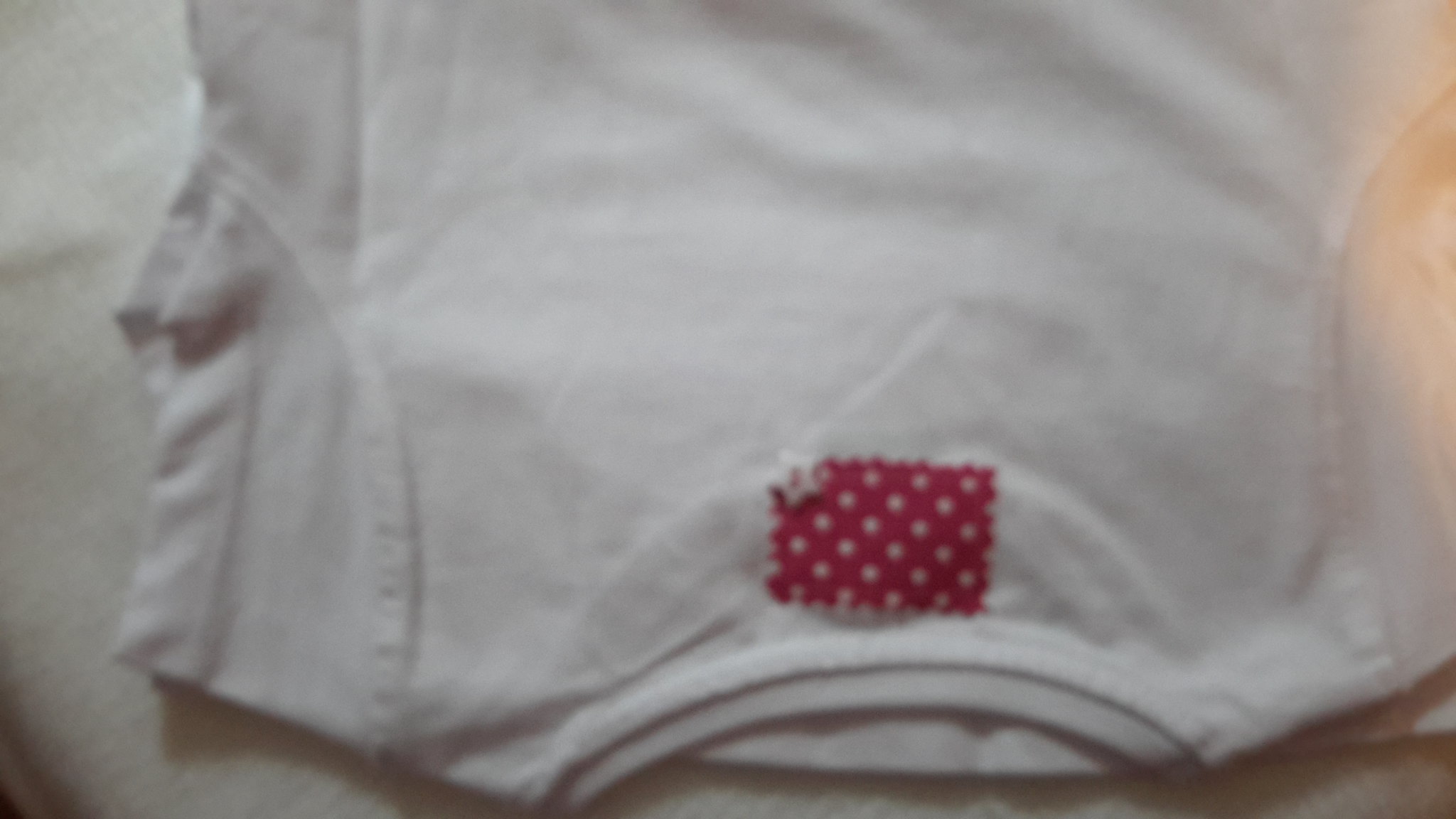An upside-down white t-shirt with partial sleeves is displayed in the image. The visible left sleeve extends to the upper arm, while the right sleeve is cut off from the frame. The t-shirt features a double-lined collar, located centrally at the top of the image. Just below the collar, a red patch with white polka dots adds a pop of color to the predominantly white garment. A light source appears to illuminate the area near the right shoulder, creating a subtle highlight. The t-shirt rests on a white background, which seems to be a piece of cotton fabric, visible especially at the far left and bottom edges of the image.